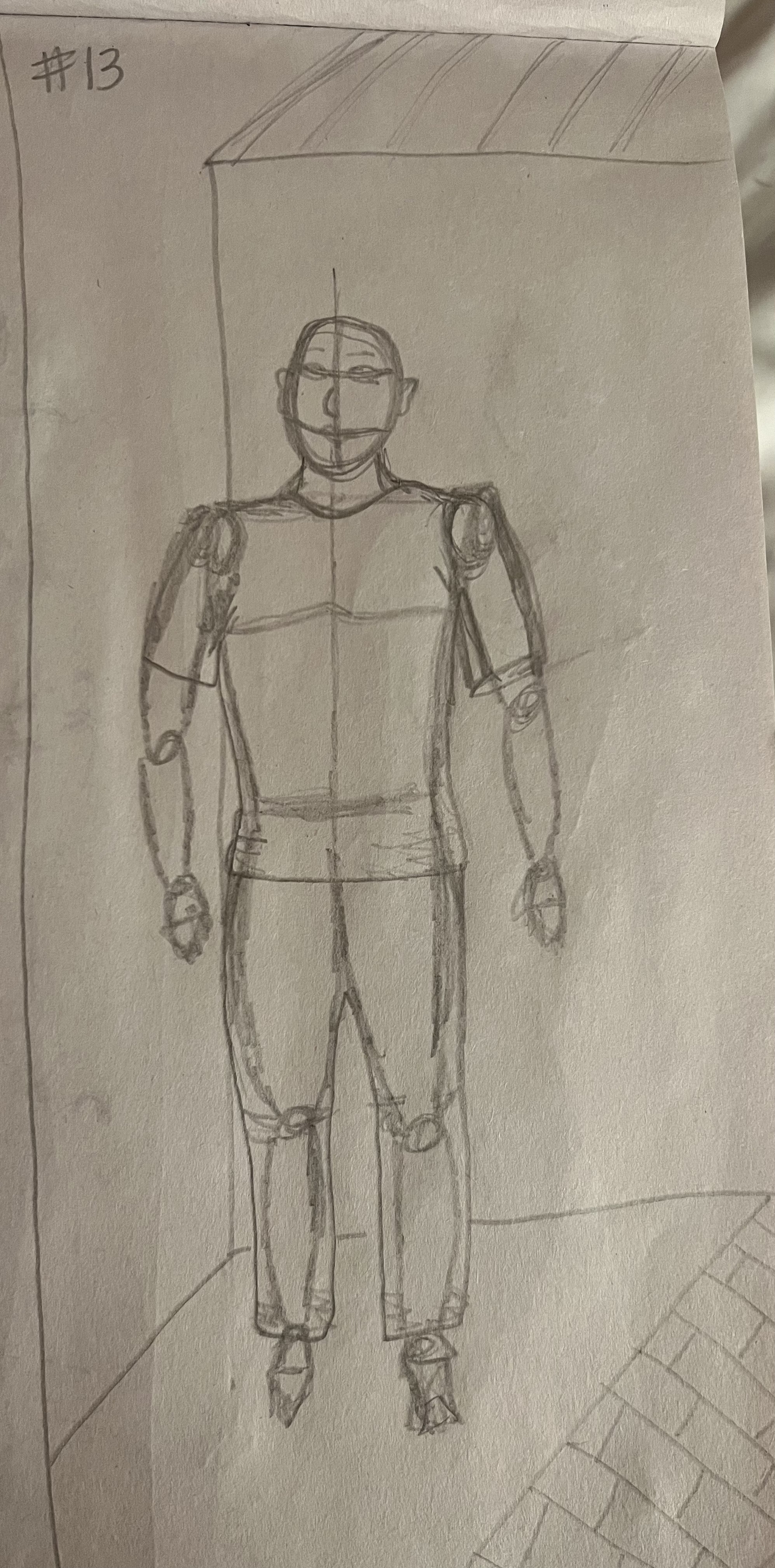The image depicts a rough pencil sketch on white paper, showcasing the preliminary stages of drawing a human figure. The figure is composed of basic shapes such as circles at the joints -- elbows, knees, ankles, and shoulders -- and simple lines to outline the limbs and torso. Notably, the figure's eyes, nose, mouth, and ears are only lightly indicated, with the eyes appearing crossed out and lacking detailed features. The figure stands on what seems to be a rooftop with a ledge and a brick wall behind it, although the sketch's roughness leaves room for interpretation about the precise setting. The number "13" is prominently written at the top left of the picture. Additionally, the drawing includes sketched clothing and panel or brick patterns at the bottom right, suggesting a room or exterior wall. The image is framed by the piece of paper itself, with hints of objects or background visible at the edges, and the entire sketch is executed using pencil, producing a monochrome effect of varying shades of gray against the white paper.